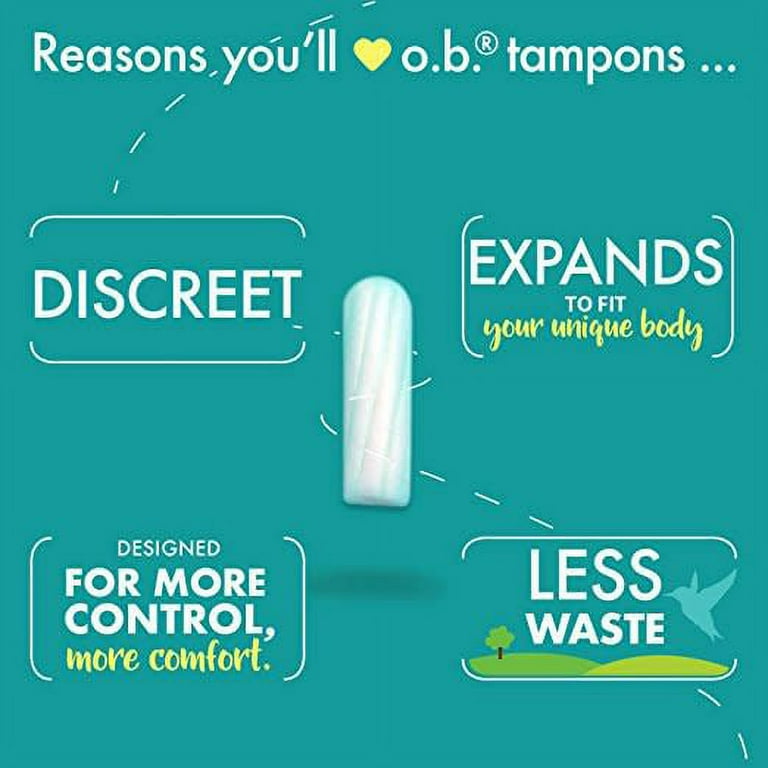This advertisement for OB tampons features a predominantly green background with white text and select accents in yellow and light blue. At the top, it says "Reasons you’ll ♥ OB Tampons," where a small yellow heart replaces the word "love." Key features are listed in bold white letters with specific highlights in yellow, including "more comfort" and "your unique body." The ad emphasizes the product's discretion, its ability to expand to fit your unique body, and its design for enhanced control and comfort. Additionally, it touts less waste, possibly due to a more compact design, as suggested by a visual of the tampon without a dispenser. Illustrative details include hills, a tree, and a bird on the right side. A depiction of the tampon is positioned centrally. The overall color scheme is a harmonious blend of green, white, yellow, and light blue, forming a clean and inviting visual appeal.